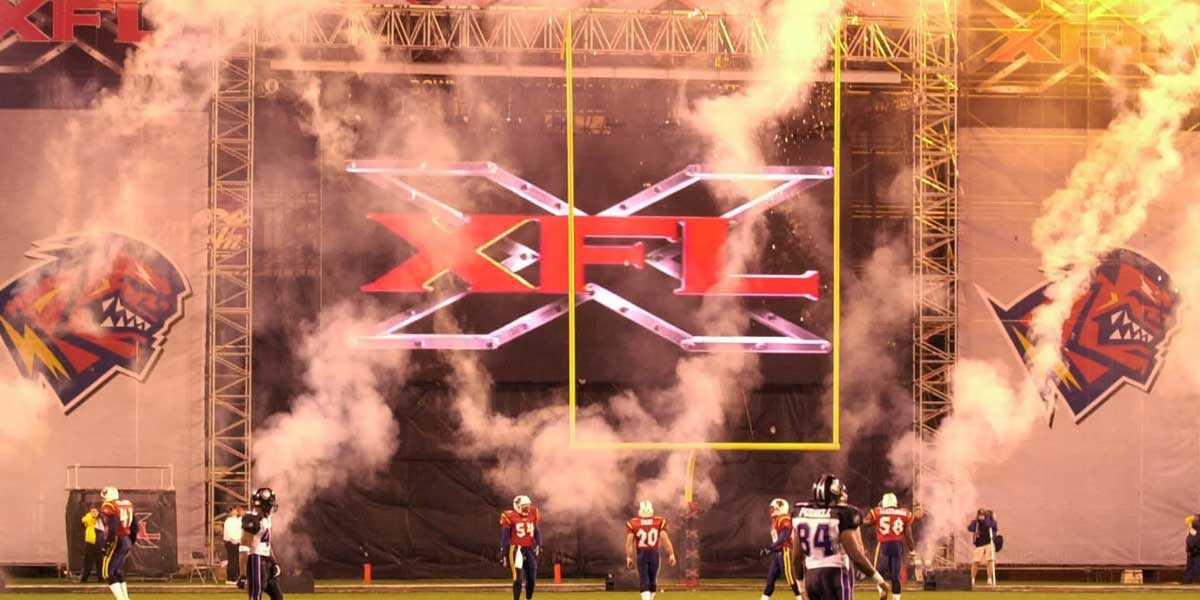This is an XFL promotional photograph taken during a live game, presented in a horizontal rectangular format. The background features a striking XFL logo in bright red letters, set against a massive black 'X' bordered by a silver metallic frame with rivet-like holes. This eye-catching logo is positioned behind a yellow goalpost. Flanking this centerpiece are large, white banners showcasing a fierce, red-faced mascot with sharp, clenched teeth and lightning bolts along its collar. The scene is further energized by smoke billowing from fireworks or pyrotechnics set off on the field.

In the foreground, a dynamic mix of players from two different teams are captured mid-action on the vibrant green field. One set of players sports white helmets, red jerseys with white numbers, and blue pants featuring yellow stripes. The opposing team members are outfitted in black helmets, and white, black, and purple jerseys with matching pants. The uniforms add a colorful contrast to the scene, embodying the intensity and competitive spirit of the game. Additionally, a referee clad in yellow can be seen in the bottom left-hand corner, overseeing the action. This vivid snapshot encapsulates the high-energy environment typical of an XFL football game, complete with dramatic visuals and team mascots adding to the atmosphere.